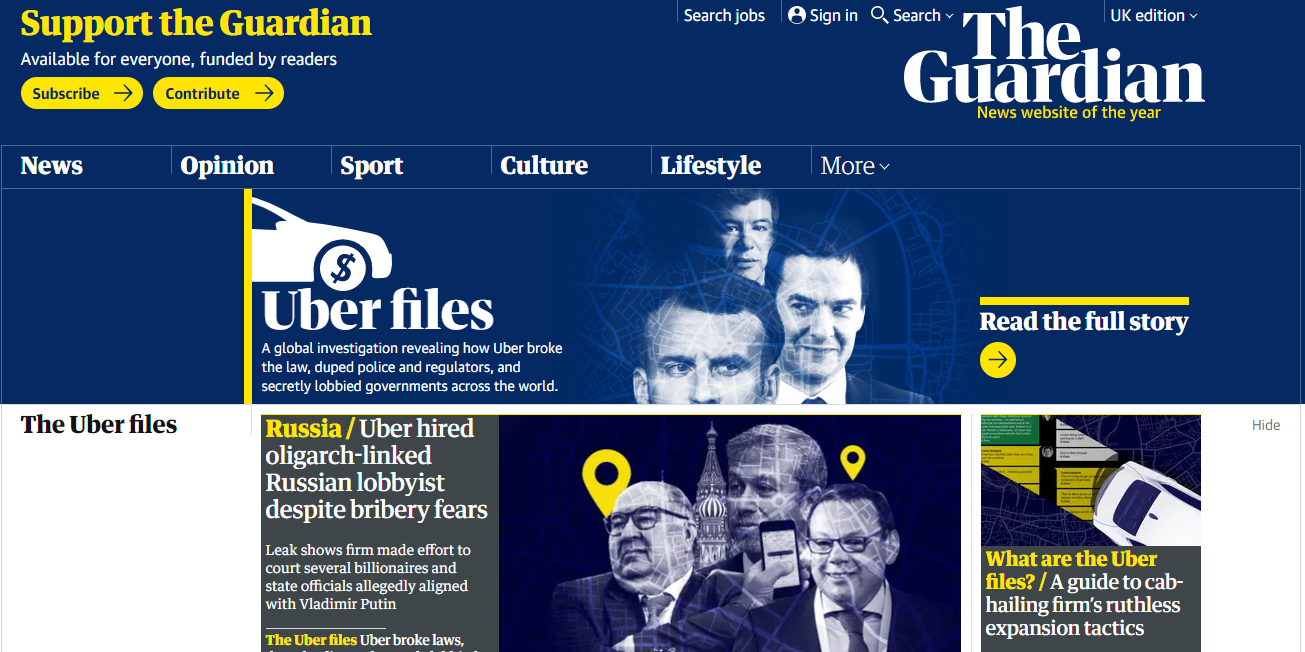The image is a screenshot set against a blue background, featuring prominently yellow and white text. In the upper left corner, it states "Support The Guardian" in white text. Below this, there's a message reading "Available for everyone, funded by readers." Two yellow action buttons are situated beneath this message: "Subscribe" on the left and "Contribute" on the right.

In the upper right corner, the publication's name, "The Guardian," is displayed in bold white block text. Beneath it, in smaller yellow text, it reads "News Website of the Year." Directly under this, there is a menu bar with the sections labeled from left to right: News, Opinion, Sport, Culture, Lifestyle, and More, with a pull-down arrow next to the last option.

The central focus of the screenshot is an icon of the front half of a car with a dollar sign on the front wheel. Below this icon, the text "Uber Files" is written in bold white font, accompanied by the description "A global investigation revealing how Uber broke the law."